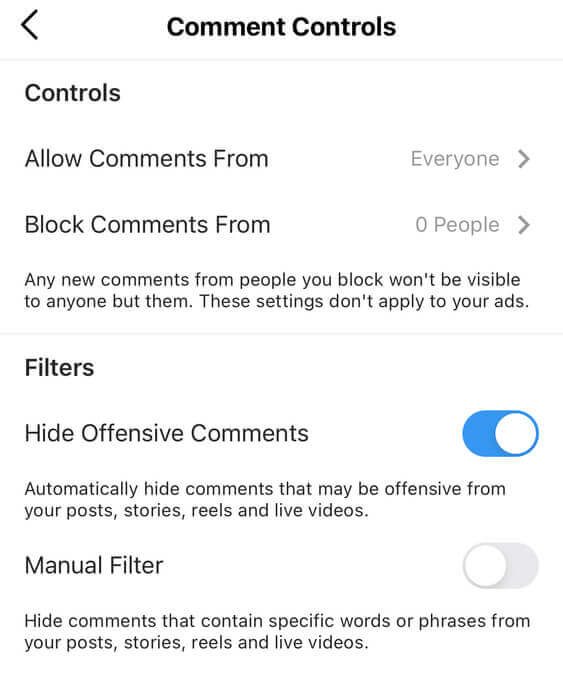In this image, the background is white with various sections of black text organized in a clear layout. At the top, the title "Command Controls" is prominently displayed in bold, black font. To the left of this title, there is a back button represented by a left-pointing arrow.

Below the title, on the left side, is a series of settings. The first line reads "Controls," followed by "Allow comments from," with the selected option "Everyone" appearing to the right. Underneath this, the text "Block comments from" appears along with the option "Zero people" displayed to the right. Clicking this option would redirect to additional choices for blocking specific commenters.

Further down, there is a note in smaller text explaining, "Any new comments from people you block won't be visible to anyone but them. These settings don't apply to your ads."

At the bottom, under the "Filters" section, there is an option to "Hide offensive comments." This setting's toggle switch is turned on, indicated by its blue and white color and rightward position. Accompanying this option is a description that reads, "Automatically hide comments that may be offensive from your posts, stories, reels, and live videos."

The final setting listed is the "Manual filter." Its toggle switch is turned off, shown by its grey color and leftward position despite being located on the right side of the text. The accompanying description explains, "Hide comments that contain specific words or phrases from your posts, stories, reels, and live videos."

The entire layout is set against a consistent white background, providing a clean and organized appearance.